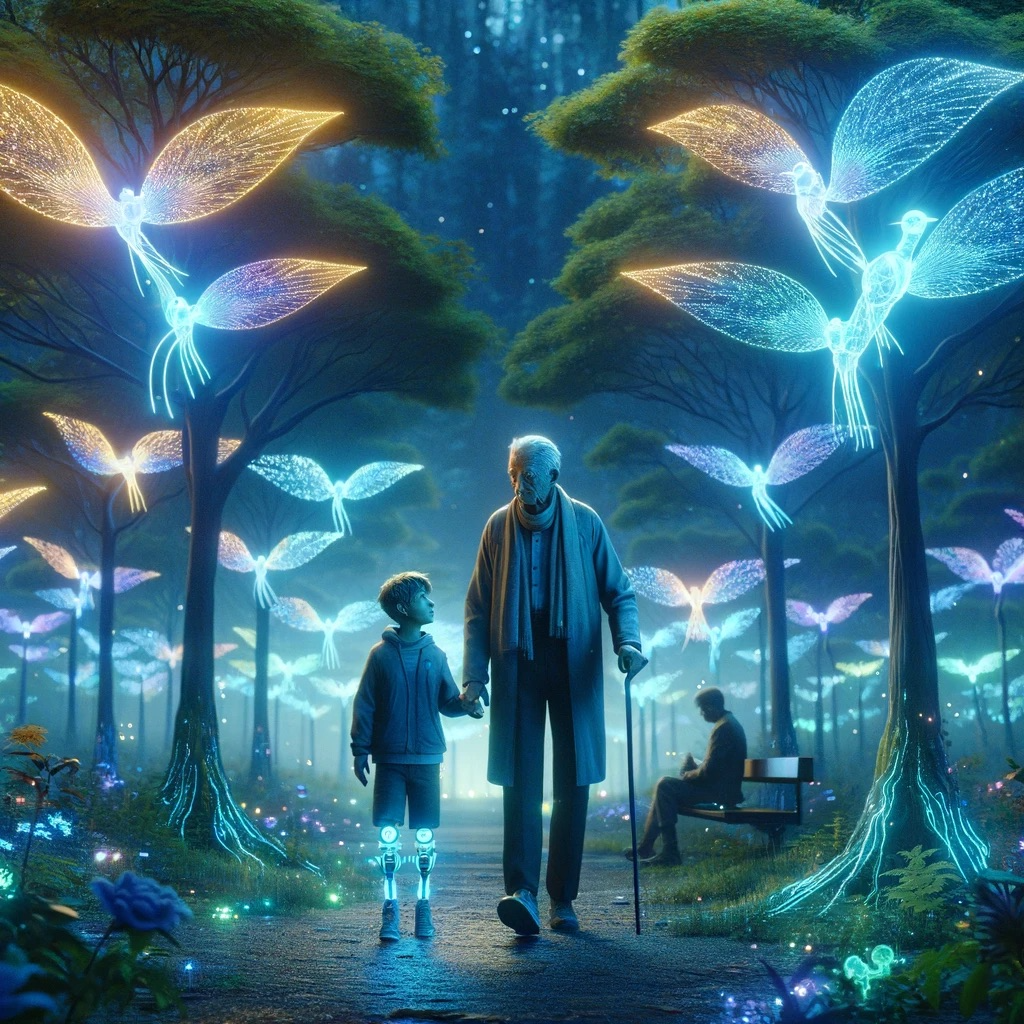In this captivating fantasy painting, a grandfather is depicted walking hand-in-hand with his grandson through a magical, park-like realm under the dim light of a night sky. The grandfather, dressed in a long jacket and scarf, uses a cane with his left hand while holding the boy's left hand with his right. The young boy, clad in a sweatshirt and shorts, has prosthetic legs from the knee down that glow with a mesmerizing blue light. The scene is enveloped in dark blues and greens, creating a whimsical contrast against the many glowing elements within the painting. Dozens of ethereal, holographic birds with luminous wings fill the sky, their radiant forms distinctly visible especially in the upper portions of the image. On either side of their path, large trees and sporadic glowing flowers contribute to the enchanting ambiance. Glowing tree roots and scattered sparkles on the ground further enhance the fantastical atmosphere. In the background, a man seated on a park bench adds an element of serene contemplation, despite the magical surroundings. The overall effect is a harmonious blend of darkness punctuated by bright, pale blue and white glows, making the scene both futuristic and otherworldly.